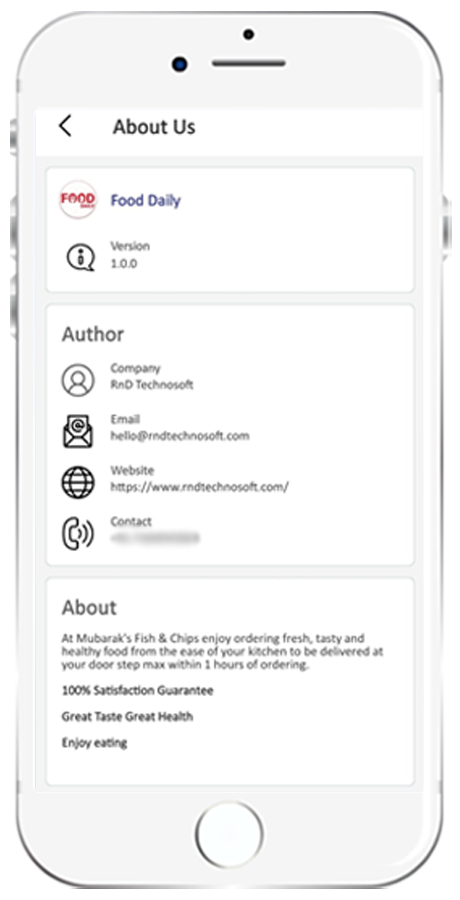The image depicts a cell phone screen displaying the "About Us" section of the "Food Daily" application. At the top of the screen, within a white rectangle, the text "About Us" is prominently featured, accompanied by a left-pointing arrow on the left side. The phone’s physical buttons, including the power button and volume controls, are visible along the edges of the device.

At the top of the app interface, the name "Food Daily" is displayed, along with a red icon featuring the word "Food" and a smaller "Daily" text tucked into the corner. Additionally, the app version "Version 1.0.0" is noted, alongside a speech bubble enclosing the letter "i."

Below this header, the section lists the author details with corresponding icons: a human silhouette for "Company," an opening envelope for "Email," a globe for "Website," and a ringing phone icon for "Contact." The specific contact information is blurred out for privacy, while the email is shown as hello@rndtechnosoft.com and the website URL is indicated as starting with "HTTPS."

Further down, the "About" section provides a description stating, "At Murr Barracks Fish and Chips, enjoy ordering fresh, tasty, and healthy foods,” with the text continuing further down the page.